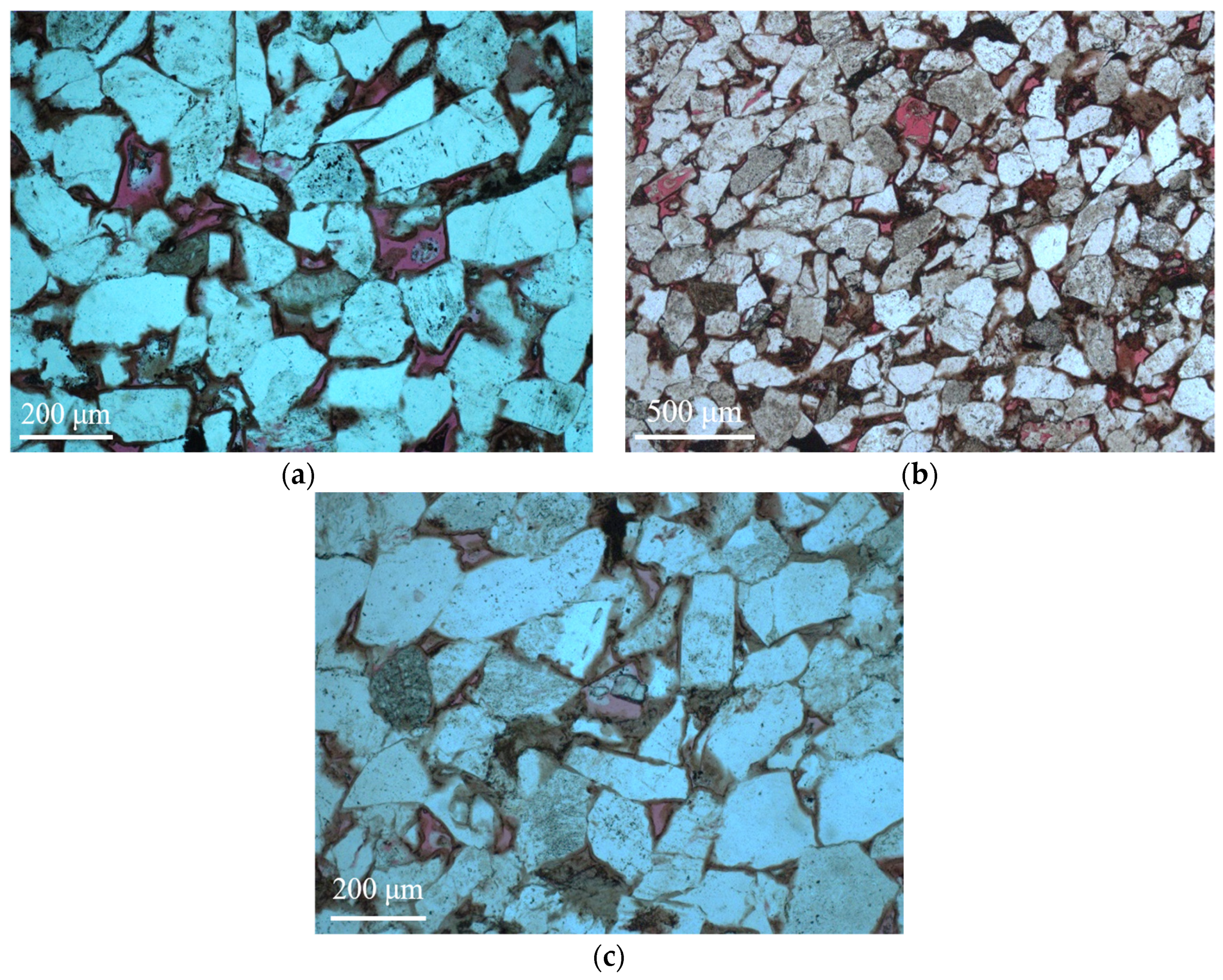The graphic features three images arranged in a two-over-one layout. The top left image, labeled "A," depicts a collection of jagged rocks in various shapes, predominately featuring a striking electric glow-in-the-dark baby blue color, along with some purple, charcoal, and black rocks. A white line at the bottom left corner is marked with "200 μm" to indicate the scale. The top right image, labeled "B," presents a different assortment of gravel-like rocks, in more neutral tones of gray, pinkish-purple, brown, white, and black. This image has a white line marked with "500 μm" in the lower left corner. The bottom center photograph, labeled "C," returns to colors similar to those in image A, though less luminous, including purple, gray, and white rocks. Similar to image A, the scale here is also marked as "200 μm," yet the rocks appear slightly larger and less defined. Overall, the images—while varying in coloration and contrast—consistently showcase different collections of gravel-like materials, providing a comparative visual of rock textures at microscopic scales.